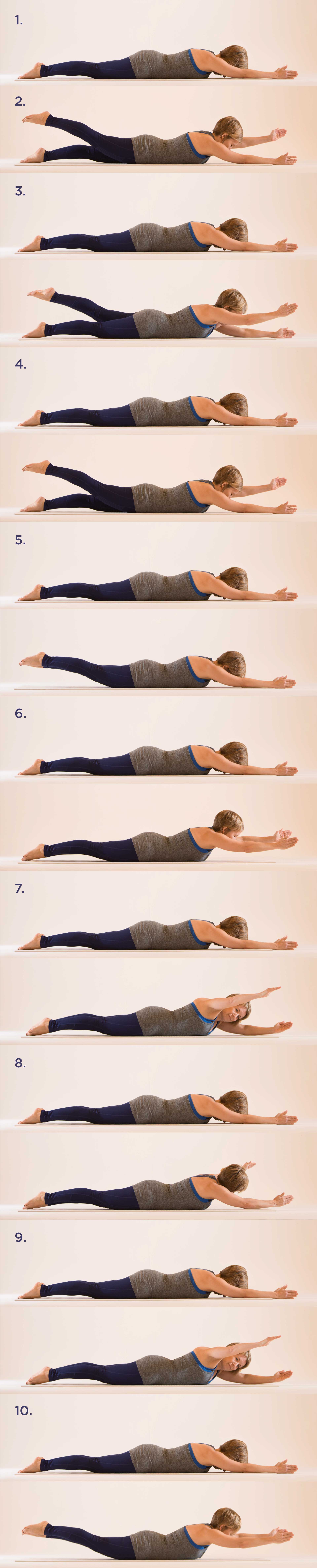This image consists of approximately 19 to 20 vertically stacked panels, out of which 10 are labeled. Each panel captures a woman performing various floor exercises. She is wearing a gray leotard with blue trim, which might be another garment underneath, paired with black leggings that have open feet, revealing her light-colored skin. The woman, who has short blonde hair, is seen lying on a floor with a peach-colored wall in the background. Throughout the series of images, she demonstrates a range of movements, including lifting her legs and raising her arms, indicative of a structured exercise routine aimed at strengthening muscles or improving flexibility.